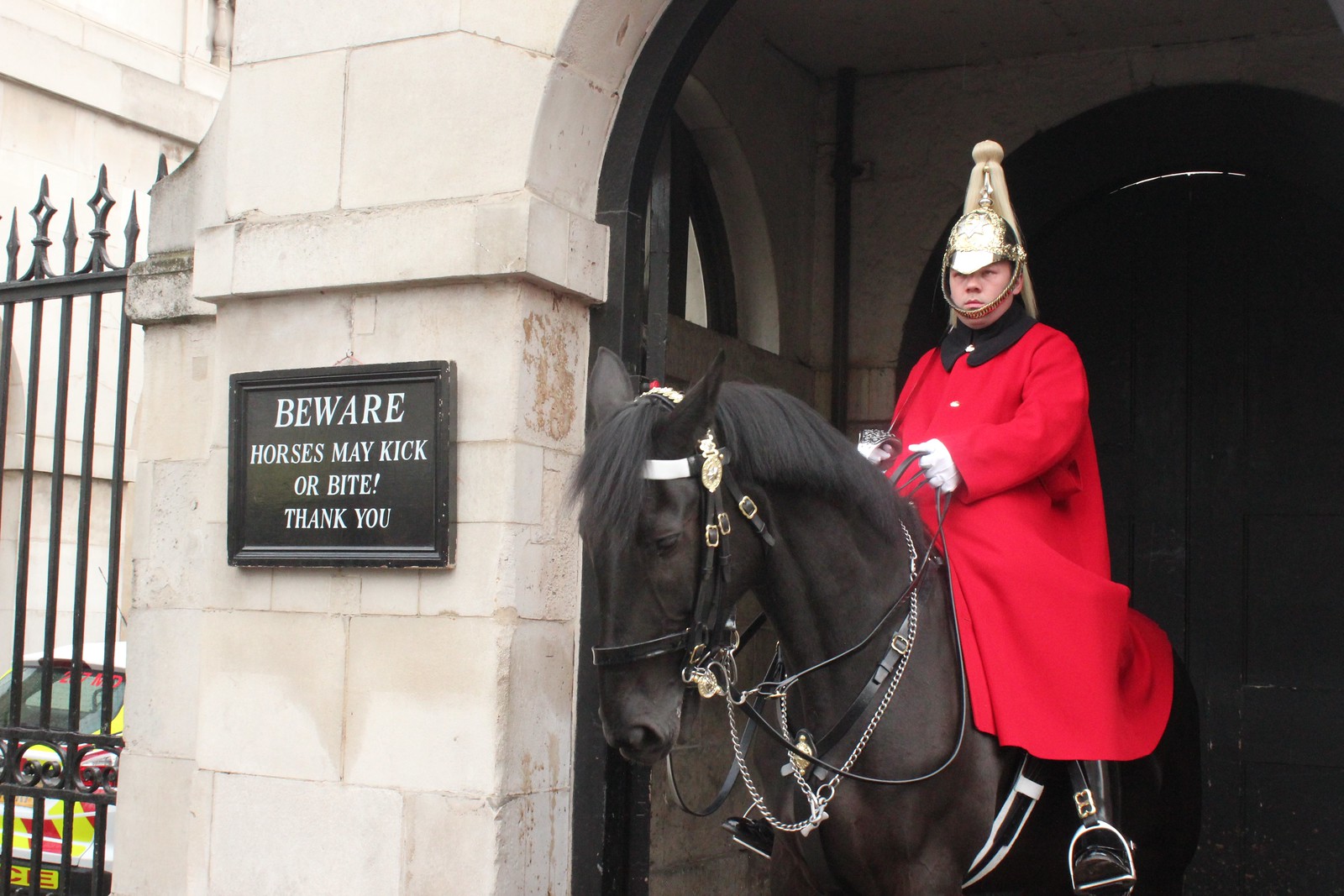The photograph captures a British cavalryman, vividly detailed, sitting atop a black horse. The scene is set outdoors, in front of a stone arched entryway of what seems to be a palace. The guard dons an elaborate gold helmet, adorned with a blonde plume, and secured with a gold chin strap. He is dressed in a striking long red coat with a high black collar and white gloves. The horse, standing calmly with its head slightly lowered and facing left, highlights the guard’s imposing presence.

To the left of the horse and rider is a tall wooden door, arched at the top, and flanked by large stone blocks forming the entryway. Adjacent to this, a black metal gate with pointed spikes is visible, beyond which there appears to be an emergency vehicle. Prominently displayed on the stone wall between the door and the gate is a black sign with white lettering that reads, "Beware: horses may kick or bite. Thank you." The photograph, seemingly taken during the daytime, captures the regal and vigilant atmosphere characteristic of British ceremonial guards.